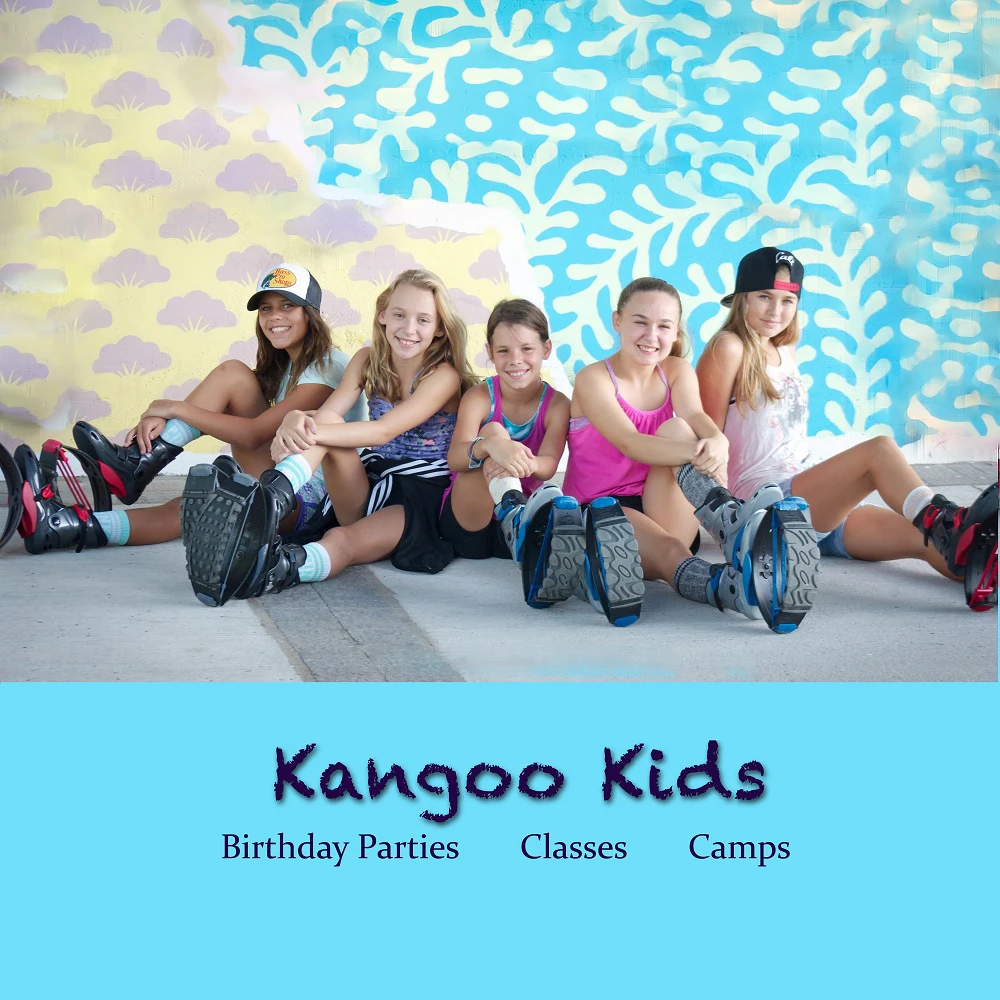The image is an advertisement featuring five light-skinned kids, consisting of two girls on each side and one boy in the center, all sitting on what appears to be a carpeted rug. The children are dressed in colorful summer attire, including tank tops in shades of pink, white, and a floral pattern, paired with shorts. They are wearing specialized boots that resemble rollerblade boots but have distinctive curved, bendable rubber soles designed for jumping or bouncing, resembling a trampoline effect. The two girls on the ends wear baseball caps—one with the Bass Pro Shop logo facing forward and another turned backward. The backdrop is split diagonally: the left side features a yellow background with puffy purple clouds, while the right side displays a blue background adorned with white leaf-like decorations. At the bottom third of the image, there's a bold blue bar with textured black text in the center reading "Kangoo Kids," followed by smaller text underneath that informs about "birthday parties, classes, camps."